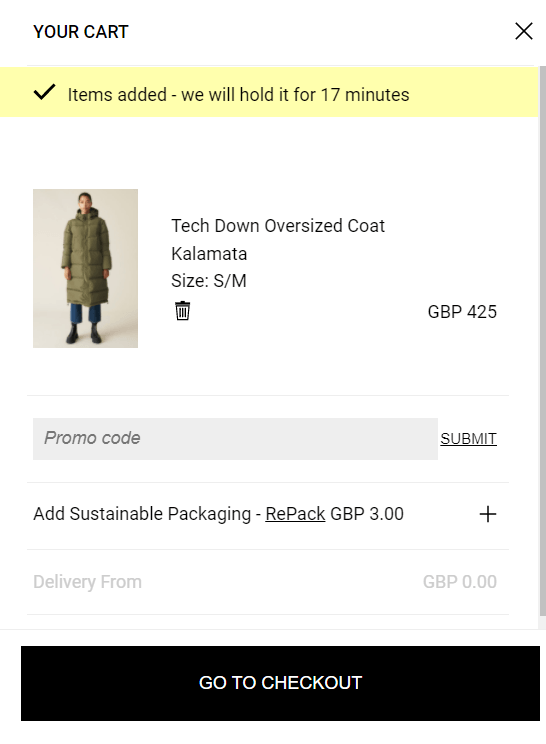The image is a mobile screenshot of the "Your Cart" section from a shopping website, set against a white background. At the upper-left corner, the title "YOUR CART" is displayed in capital letters, while an 'X' symbol for closing the cart appears at the top-right corner. Directly below the title, a pale yellow banner with a black checkmark indicates that the items have been added to the cart and will be held for 17 minutes.

Within the cart is a listing for an item featuring a woman modeled in an oversized, olive green, puffy coat named "Tech Down Oversized Coat, Kalamata." The woman, facing the camera, wears blue jeans and black shoes with her hands casually resting by her sides. 

Beneath the item description, a trash icon provides the option to delete the item. The displayed price of the coat is GBP 425.00. Further down, a gray text box labeled "Promo Code" with an underlined "Submit" button allows customers to enter a promotional code.

Additionally, there is an option to add sustainable packaging for an extra GBP 3.00, marked with a plus sign on the right. Below this option, pale gray text reads "Delivery From," with a grayed-out price of GBP 0.00.

At the bottom of the screen, a large, black "Go to Checkout" button is prominently placed. The screenshot also features a thin gray vertical scroll bar on the right side of the screen, indicating more content is available to scroll through.